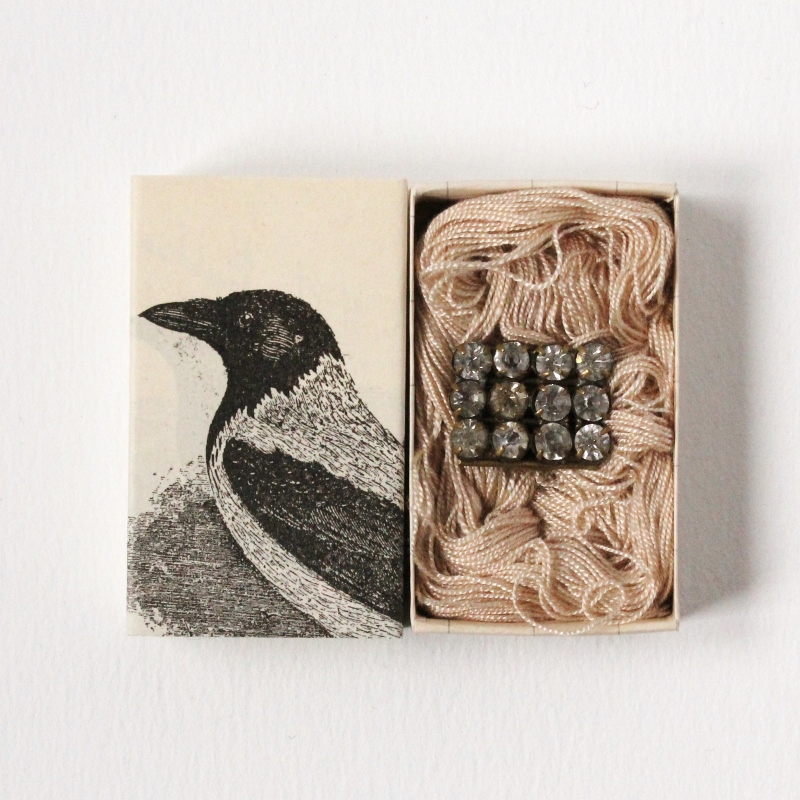In this detailed photograph, we see an open box with its lid placed to its left. The lid is adorned with a professional black-and-white sketch of a raven in a side profile, facing left. The raven has a distinctive appearance with a black head, white back, a black wing, and a white belly. Inside the box, there is a skein of thin, pinkish-beige yarn neatly arranged. Centered on top of the yarn is a smaller square box featuring a grid of gemstones, laid out in four columns by three rows, appearing as diamonds or rhinestones. The box and its contents rest on a plain white background, highlighting the intricate details of both the bird sketch and the shimmering gemstones.